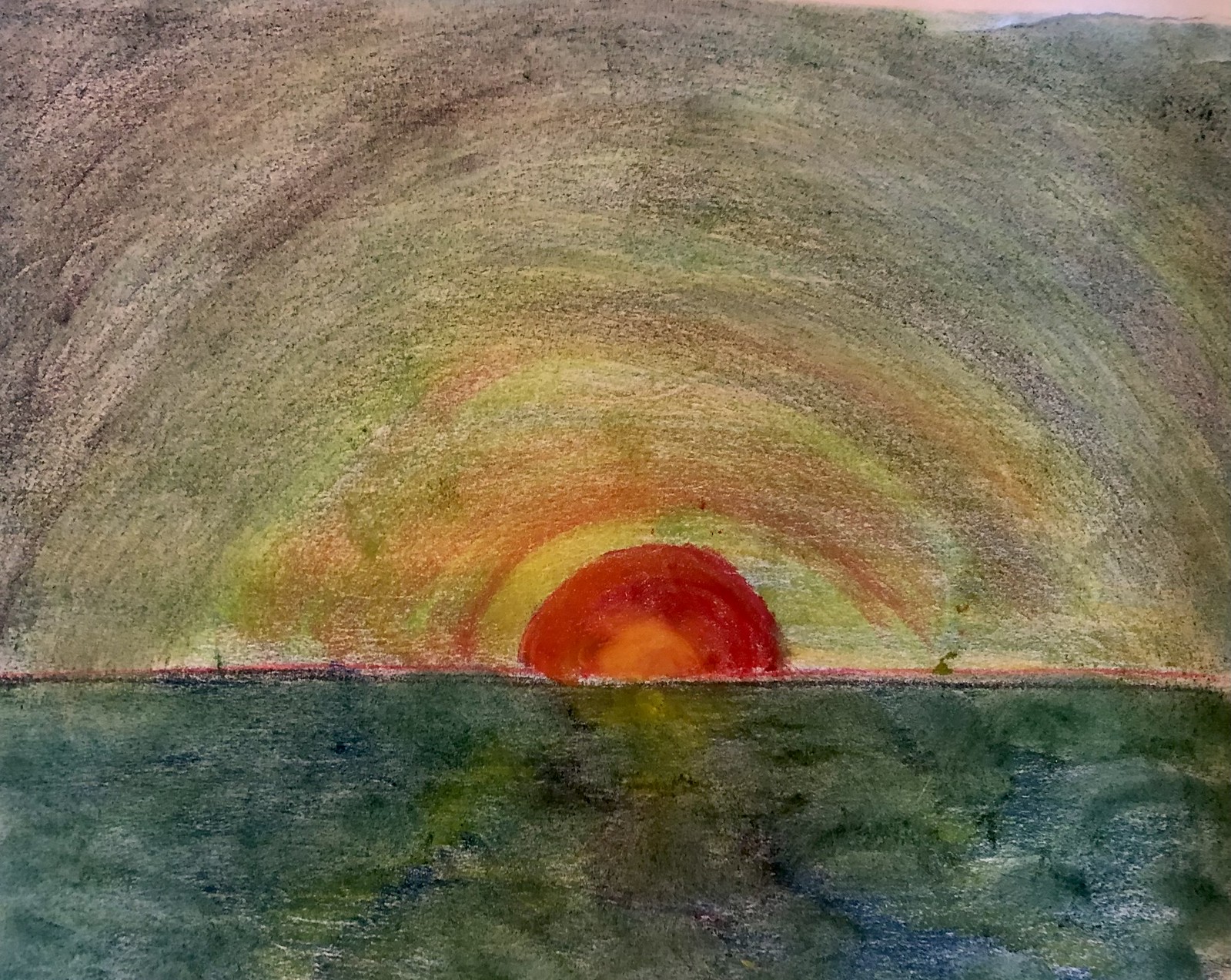A striking drawing or painting depicting a captivating sunset over a waterfront. The rich color palette includes an array of blues, greens, yellows, reds, blacks, and pinks, merging to create a mesmerizing scene. The bottom third of the image represents the water, featuring a harmonious blend of blues, greens, and yellows. The yellow hues intensify closer to the sun, highlighting the transition from water to sky. In the sky, the sunset is illustrated by a prominent red circular area at its center, surrounded by varying shades of orange, red, and yellow that radiate outward in a semicircular pattern. These vibrant colors gradually shift to green and eventually to gray, capturing the serene yet intense beauty of the setting sun.